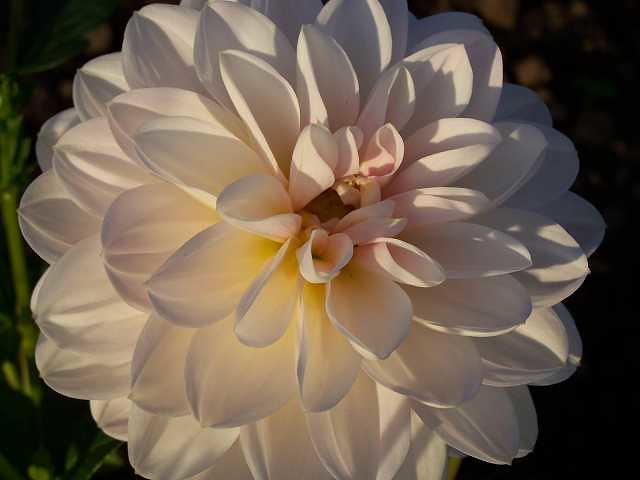This zoomed-in image captures a captivating white flower, filling the entire frame to the extent that the top and bottom portions of the flower are slightly cut off due to its large size. The petals are arranged in a perfect circular fashion, with multiple rows contributing to its intricate structure—one can count approximately 10 petals in just the second row alone, with five or six rows in total, making for a highly detailed appearance. The flower's center subtly transitions from a faint pink to a yellowy hue, adding depth and color variation. Illuminated from the bottom left, the lighting casts beautifully aesthetic shadows, particularly on the right side, enhancing the flower’s detailed texture and making the white petals stand out vividly against the black background. The absence of the flower’s stem or center further accentuates its surreal, almost otherworldly perfection.